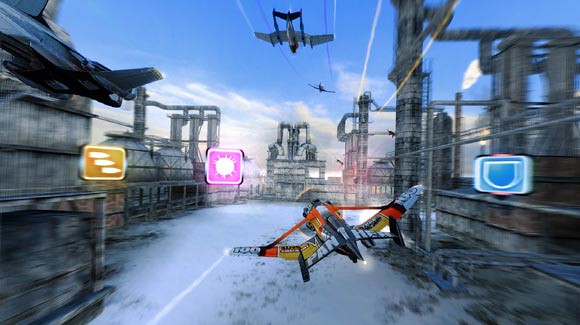This screen capture from an action-packed, futuristic video game presents a landscape-oriented scene of sleek, first-person perspective aircraft zooming through an industrialized, dystopian urban structure. Dominating the scene is a brightly colored plane, close to the viewer, with striking orange and yellow highlights accentuating its gray body, leaving an exhaust flame in its wake. Other planes, purely gray, follow the same high-speed path through the metallic labyrinth of buildings that stretch into the blue sky. Central to the image are three prominent icons: a pink square with a starburst pattern, a detailed orange square featuring bullet symbols, and a blue square depicting a shield. This vibrant, busy snapshot captures the thrilling essence and rapid pace of the immersive gameplay.